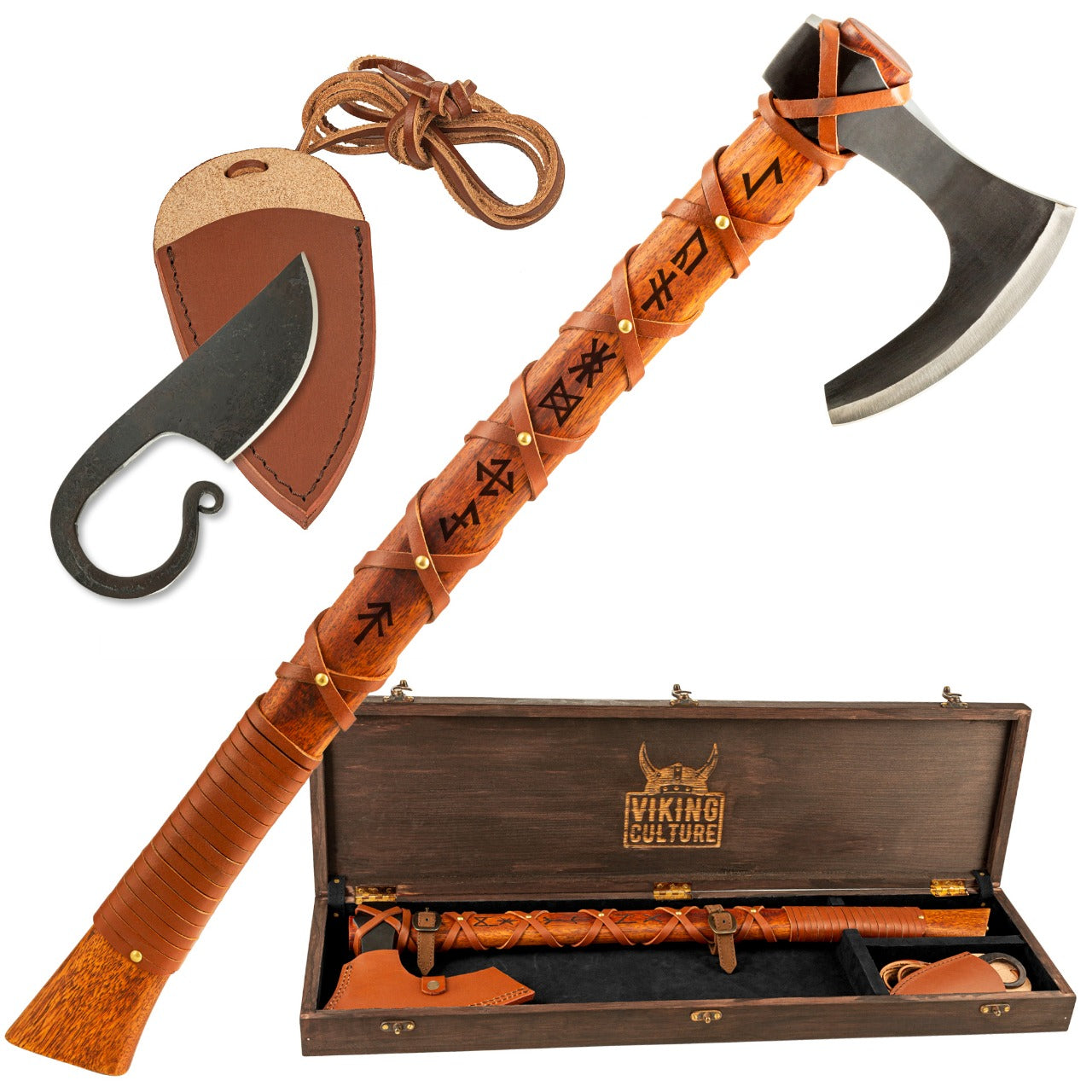This detailed product image showcases a bespoke wooden box emblazoned with the words "Viking Culture" and an etched Viking helmet on the inside of the lid. Within this rustic wood grain box with a dark wood and black velvet backing, two Viking implements are prominently featured. The first is a single-headed Viking axe, marked by its wooden handle intricately adorned with burned-in Nordic runes running down the center, and a black and silver blade secured with leather straps that provide a sturdy grip. Accompanying the axe is a small, sharp knife with a hilt that elegantly curves into the handle. The knife is paired with a matching leather-bound sheath, fitted with a leather cord for easy attachment. Adjacent to these items in the box are a detailed depiction of the axe outside the box and the knife in the leather sheath, offering a comprehensive view of these meticulously crafted Viking tools.